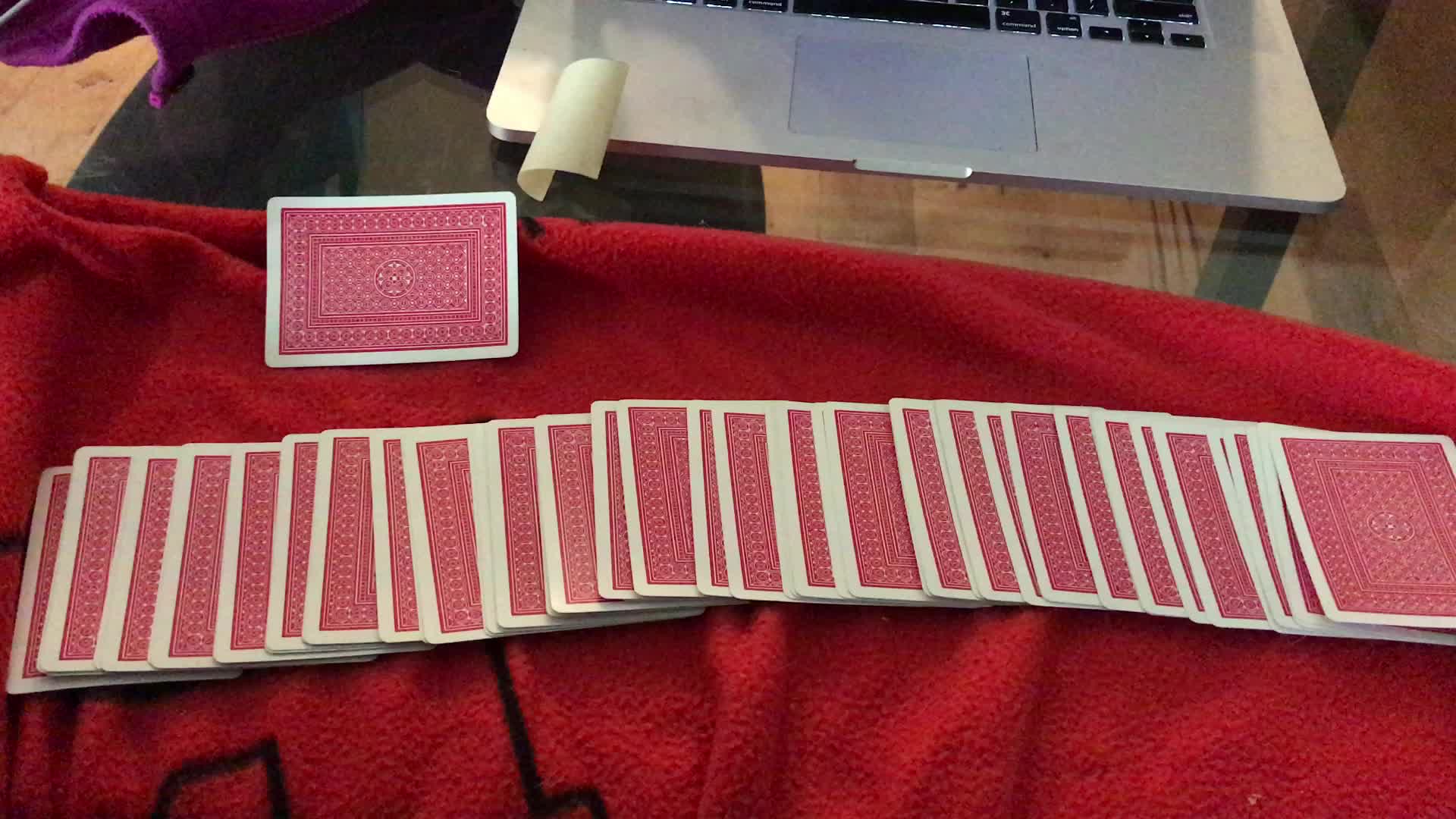An aerial view captures a desktop setup featuring what appears to be an Apple Mac computer, identifiable by its distinctive keyboard design. A partially folded yellow sticky note is affixed to the screen, obscuring any written content. In the foreground, a vibrant red fabric—likely a blanket or towel—serves as a backdrop for an array of playing cards scattered across its surface. The cards, numbering around ten, are predominantly red with white borders. Additionally, a curved black object, possibly a shoestring, weaves through the scene, adding a subtle element of intrigue to the composition.